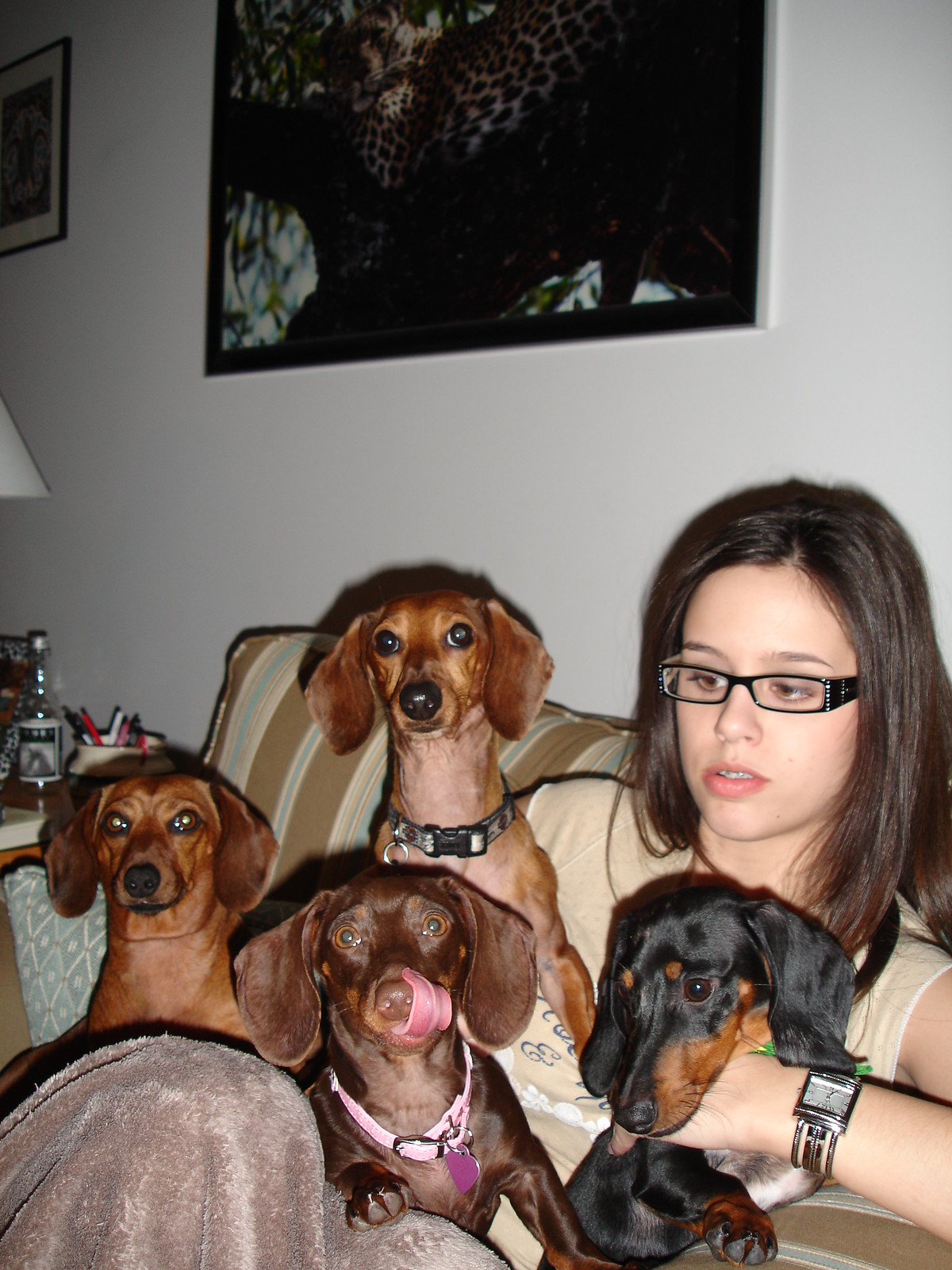In this detailed photograph, a woman is sitting on a striped couch with brown and blue stripes, slightly slouched, with her shoulder-length dark hair parted in the center. She wears black-rimmed spectacles with a bejeweled edge and has a brace on her teeth. A silver square watch adorns her left wrist. Draped across her lap is a light brown fuzzy blanket, and nestled comfortably on her lap are four miniature dachshunds. Three of the dachshunds, varying in shades of brown, have their eyes fixed intently on the camera, with the middle one playfully licking its face. The fourth dachshund, predominantly black with some brown on its muzzle, gazes downward, and the woman’s gaze follows in the same direction as if they have both noticed something intriguing. In the background, a white wall is decorated with a painting of a leopard directly above the woman and another, indistinct picture on the top left. To the side of the couch is a table holding a pot of pens, a bottle of liquid, and the shade of a lamp can be seen intruding from the left side of the frame.